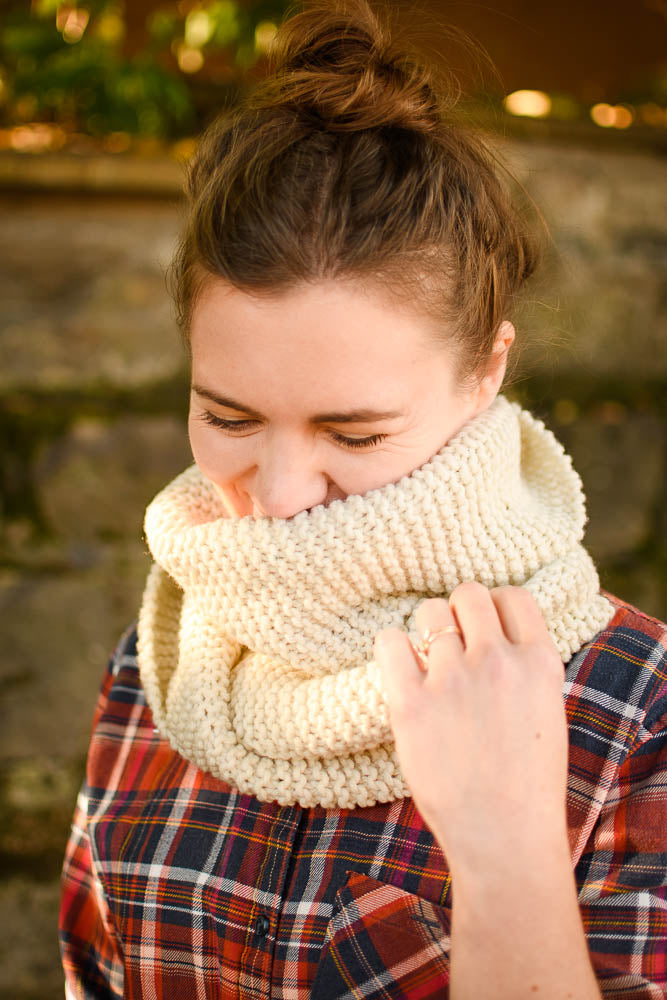This color photograph captures a close-up, head-and-shoulders view of a Caucasian woman with brown hair, which is elegantly twisted up and slightly messy on top of her head. Her eyes are closed, or she is looking down, and she appears to be smiling subtly beneath a large, knitted off-white (or tan) wool scarf that covers her neck, mouth, and most of her left cheek. She is dressed in a flannel, plaid button-down shirt with rolled-up sleeves, revealing part of her wrist. Her left hand, bent upward, touches the scarf and prominently displays a gold ring on her ring finger, possibly a wedding ring. The background is softly out of focus but suggests the presence of a brick wall, plants or trees, and small lights bedecked by sunlight shining on her.